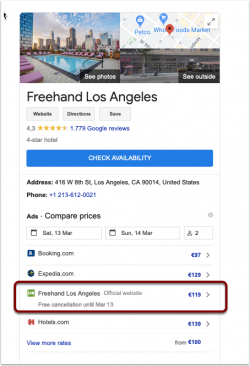This is a cropped screenshot likely captured from a cellphone given its narrow, portrait orientation. The predominantly white background includes various text and image elements. At the top left, a thumbnail image showcases a cityscape background with a pool and several deck chairs in the foreground. To the right, a second thumbnail image includes a map at the top and a photograph of a location sourced from Google Photos beneath it. 

Centered below these images, bold text reads "Freehand Los Angeles." Directly beneath this text are three small, grey buttons whose information is illegible due to their size. Below these buttons, the image displays a rating of 4.3 stars based on 1,779 Google reviews.

Next, a blue button spanning the image width bears the text "Check availability" in white. Under this button, the word "Address" is followed by the specific location and a blue, clickable phone number for direct calling capabilities.

Further down, there is a section labeled "Compare prices," featuring options to input dates and view price comparisons from Booking.com and Expedia.com. One selection titled "Freehand Los Angeles" is highlighted by a maroon circle, indicating the user's choice. 

Finally, another website is mentioned at the bottom, but its text is too small to decipher clearly.